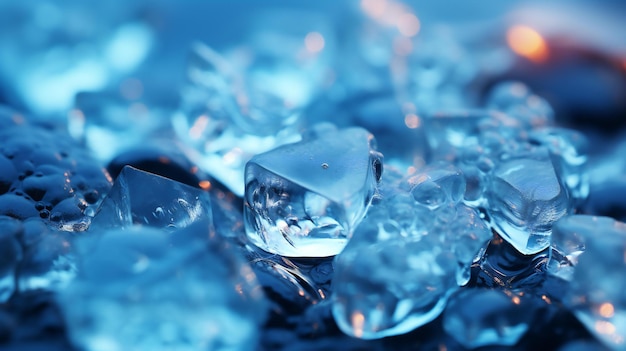The image is a highly detailed, close-up photograph featuring clear crystalline structures that appear to be either ice or some sort of broken glass. The focus varies, with only a few of these transparent pieces clearly in focus, while others in the background blur out. The entire image is tinted with blue light, creating various shades from dark to light blue across the scene. There's a reflection from a light source, possibly the sun or an overhead light, adding a prismatic effect to some parts of the image.

In the foreground, these clear chunks with smooth surfaces resemble ice blocks, though they could also be small pieces of glass or crystals found in nature or made in a laboratory. These pieces are set against a black, glossy, and somewhat reflective surface that resembles obsidian. On the left side of the image, there are water droplets and black, oily bubbles. In the upper right corner, a large black oval shape stands out against the blue background, adding to the complexity of the scene. The overall aesthetic is both mesmerizing and ambiguous, capturing the viewer’s curiosity about the true nature of the materials depicted.